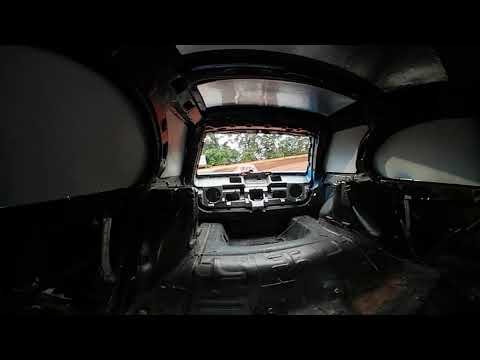The image is a detailed photograph of a gutted SUV or bus-like vehicle, framed from the perspective of someone inside the structure. The vehicle's windshield is missing, revealing a view of a tan colored building and lush green trees behind it. Inside, the car is completely stripped, with all seats, interior fixtures, electronics, steering wheel, and gauges removed. The walls and ceiling are a light gray, contrasted by dark-colored support framing throughout. The vehicle's floor is a heavily indented black metal, and small patches of various colors like blue, red, pink, and orange appear scattered across the interior. There is a rectangular window in front, around a couple of feet high and approximately four feet wide, offering a clear view of the outside landscape. Although the photo does not include any people or text, the wreck offers a stark and vivid portrayal of the stripped-down, framed vehicle amidst a serene outdoor background.